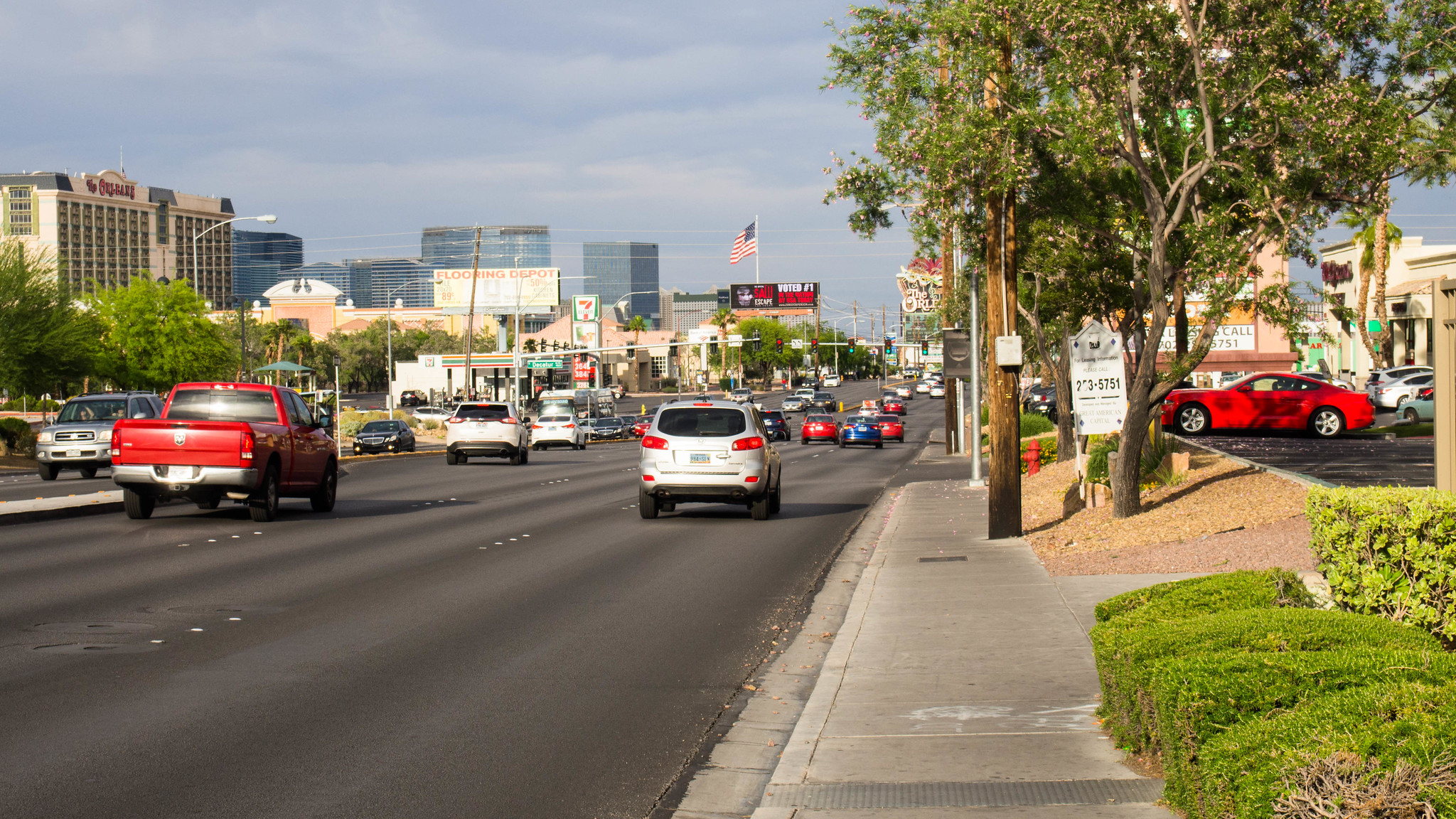The photograph captures a bustling urban scene, viewed from a vantage point overlooking a wide, multi-lane street. The street features three lanes of traffic on either side, separated by a median. At the intersection, green lights guide the cars moving away from the viewer. The area is densely built, with various edifices lining both sides of the road.

On the left side of the image, a prominent building stands out with its tall stature and numerous windows. It boasts a stylish mansard roof, suggesting it's perhaps a casino. A flag at half-mast flutters atop this building, which appears to bear the name "The Orleans," though it's not entirely clear. Adjacent to this structure is another building marked by its unique roofline, characterized by decorative columns topped with spherical ornaments.

In the background, modern high-rises constructed from glass and steel dominate the horizon, adding a contemporary touch to the cityscape. Across the street, a slightly obscured billboard promotes "Flooring Depot," its clarity diminished by the bright sunlight. Further to the left, a 7-Eleven convenience store and gas station serve the local traffic.

Directly ahead, a billboard proclaims in white text, "voted number one," and, though partially blurred, red text accompanies the message. Another sign on the right side of the street confirms the presence of "The Orleans" nearby. A parking lot behind the sidewalk on the far right contains a red sports car among other vehicles and buildings typical of strip malls.

The overall scene is relatively calm, with light traffic traversing the wide street under an overcast, blue sky.